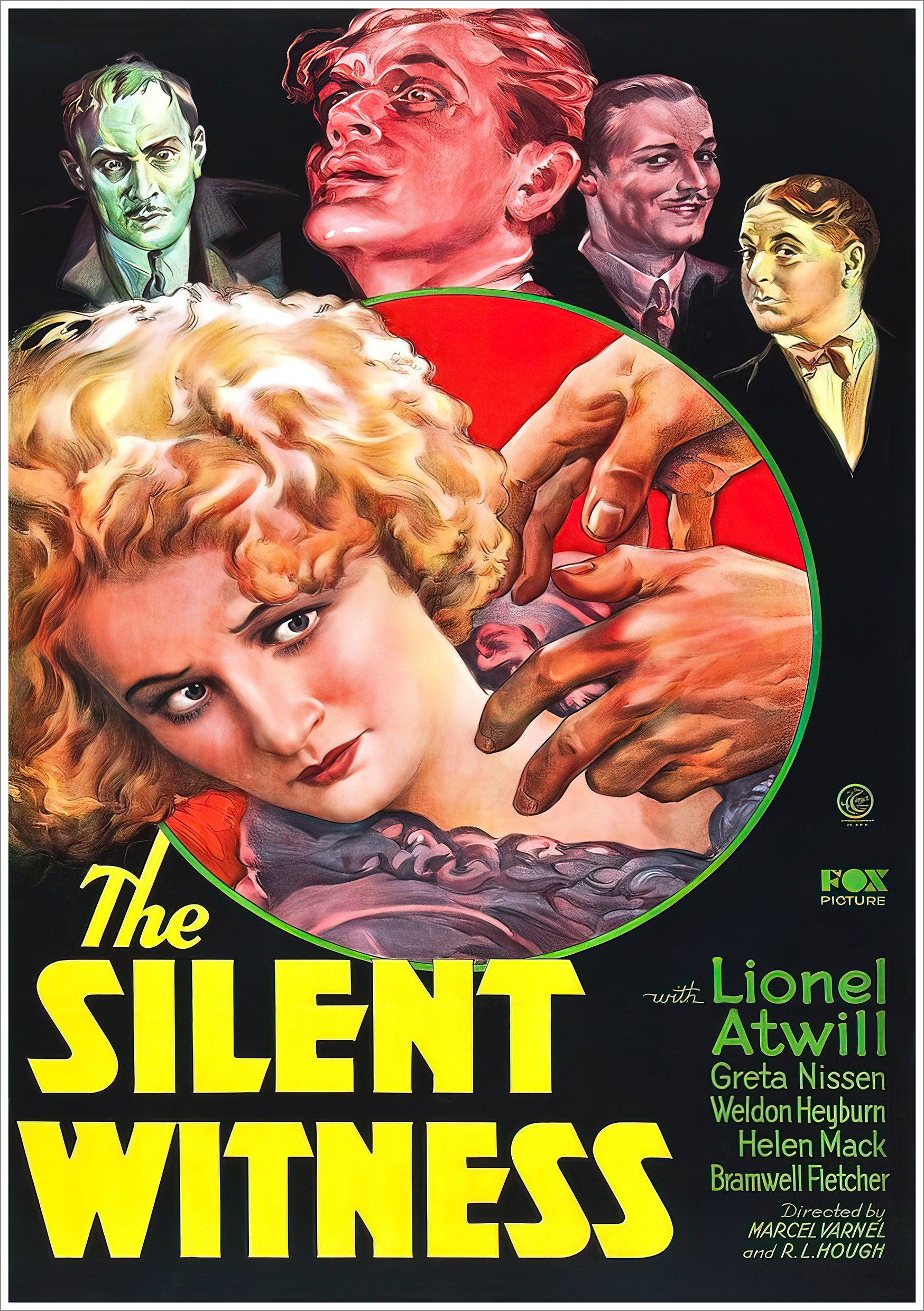This vintage poster for a classic film or play titled "The Silent Witness," produced by Fox Picture, features bold, large yellow text for the title. In the center of the poster, there is an image of a blonde woman with a frightened expression, wearing a ruffled dress, and only visible down to her bust. Her head emerges from a red circle, and a pair of hands appears to be grabbing toward her neck, suggesting a scene of potential strangulation. Surrounding the central image of the woman, there are profiles of four men at the top of the poster, each shaded in different colors: green, red, purple, and yellow. The green-hued man looks disheveled, the red-tinted man appears triumphant, the purple-shaded man is smirking, and the yellow-toned man looks perplexed. These men might be witnesses, suspects, or involved in the narrative. At the bottom right of the poster, written in lime green text, are details of the film, listing the cast members—Lionel Atwill, Greta Nissen, Weldon Heyburn, Helen Mack, and Bramwell Fletcher—and the directors, Marcel Warnal and R.L. Ho. The Fox Picture logo is also present towards the right side of the image.